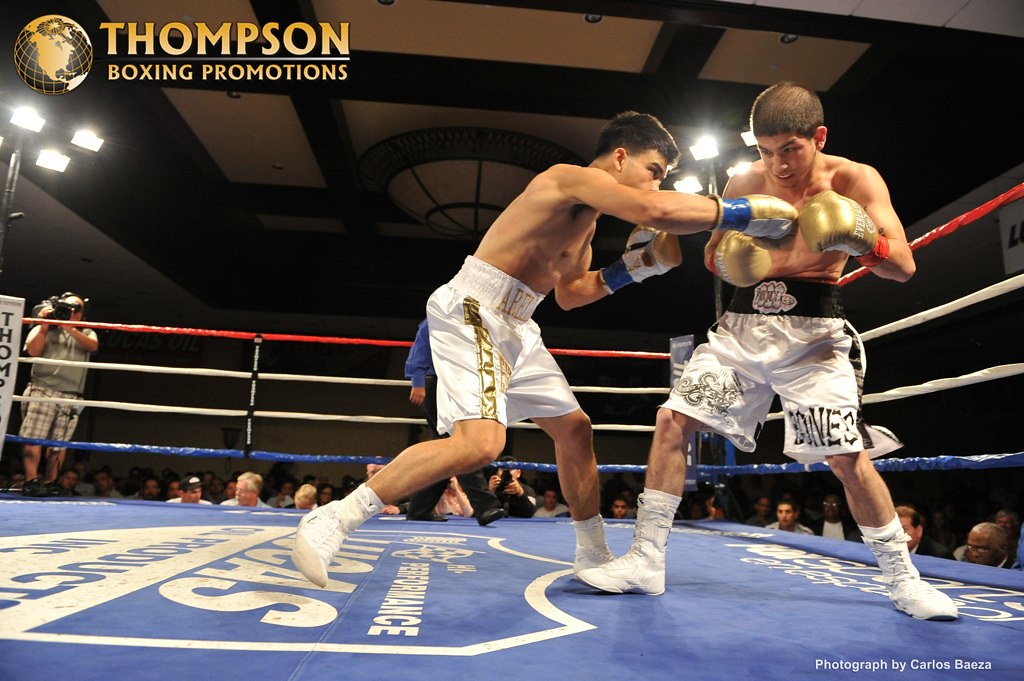This indoor photograph, approximately 6 inches wide and 3 to 4 inches tall, captures an intense moment in a boxing match promoted by Thompson Boxing Promotions. In the upper left corner, the company logo, featuring a stylized globe with the North American continent, is prominently displayed along with the promotional text. The scene is set on a blue mat with white, slightly obscured lettering, surrounded by four ropes colored red at the top, white in the middle, and blue at the bottom.

Two young boxers, likely in their mid-20s, engage in a fierce bout in the right half of the ring. Both fighters are shirtless, donning white trunks with distinctive golden embellishments. The boxer on the left, with gold writing across his waist and gold stripes down his sides, delivers a punch with his right arm, connecting solidly with his opponent's chest. He wears golden gloves trimmed with blue bands. His opponent, sporting white shorts with a black waistband and the name "Bones" emblazoned on the front, counters with golden gloves marked by red bands around the wrists. Both fighters wear white boxing boots.

The surroundings include a visible audience, seen from the shoulders up, and a refereed figure dressed in a blue shirt and black pants, partially hidden in the background. A videographer, positioned on a platform to the ring's left, documents the event. The upper half of the photograph reveals a mostly black ceiling, adding a stark contrast to the vibrant scene below. The lower right-hand corner credits the photographer, Carlos Beza (B-A-E-Z-A).